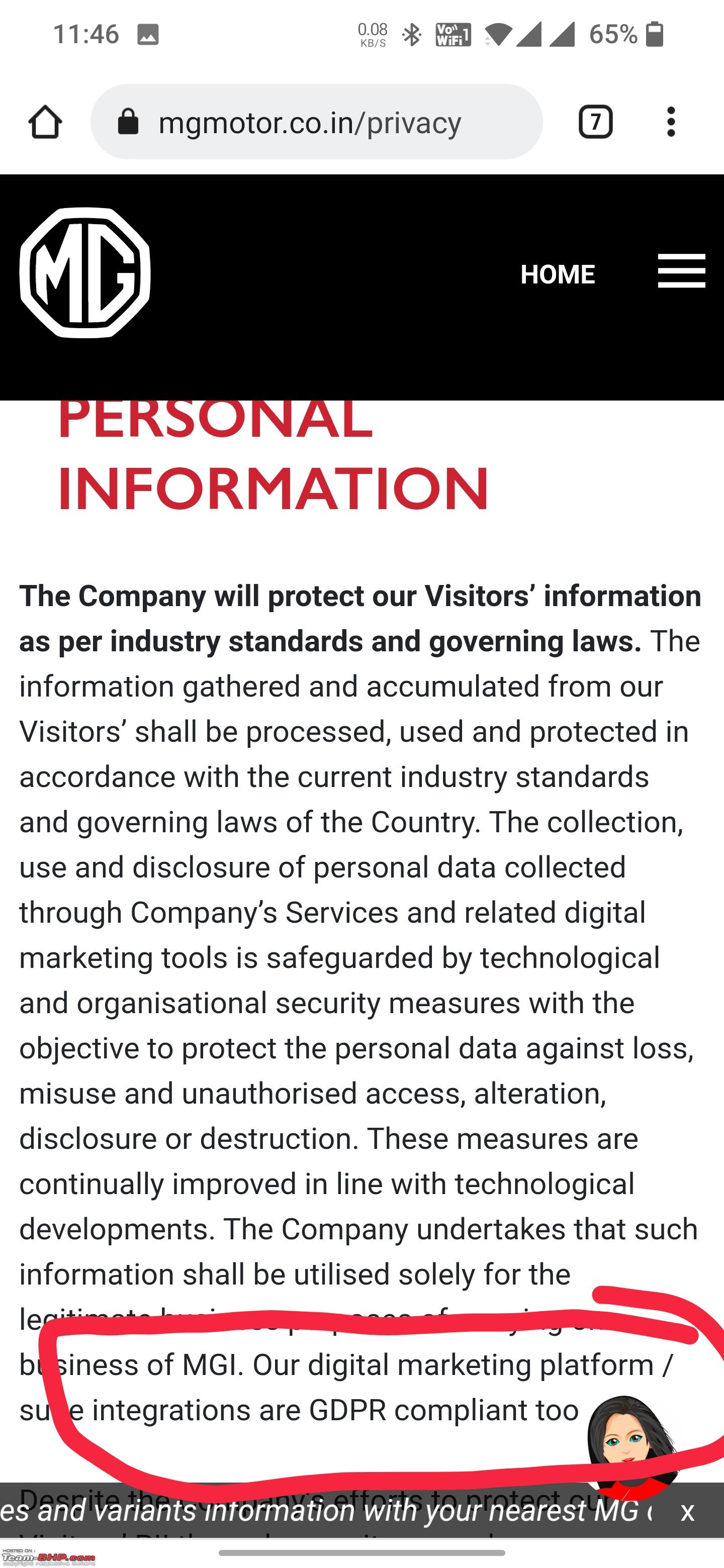In this image, the background at the top is pure white. The time displayed on the screen is 11:46, and the device shows several icons alongside a 65% battery indicator. There is an up-arrow icon, followed by a gray box containing the text "mgmotor.co.n/privacy." 

There is a square icon with the number seven, accompanied by three dots. Below this, a large black box features prominently, housing a smaller white box with the text "MG" in white. Below "MG," the word "Home" is displayed, along with three small horizontal marks.

The text within the black box is structured with the heading "Personal Information" in red. Following this, in black text on a white background, there is detailed information about the company's commitment to protecting visitor information according to industry standards and governing laws. The text elaborates on the collection, usage, and safeguarding of personal data through company services and digital marketing tools, mentioning the implementation of technological and organizational security measures. These measures are stated to be continuously improved to protect against unauthorized access, misuse, and loss of data.

The statement ends with an unfinished sentence, "The company undertakes that such information shall be utilized solely for the..." followed by a notable red mark encircling this section. 

Additionally, the document mentions that MGI's digital marketing platform integrations are GDPR compliant. Towards the bottom, a small black strip includes the text "in variance information with your nearest MG." To the right side of the image, there is a photograph of a woman with black hair and a white 'X' over her.